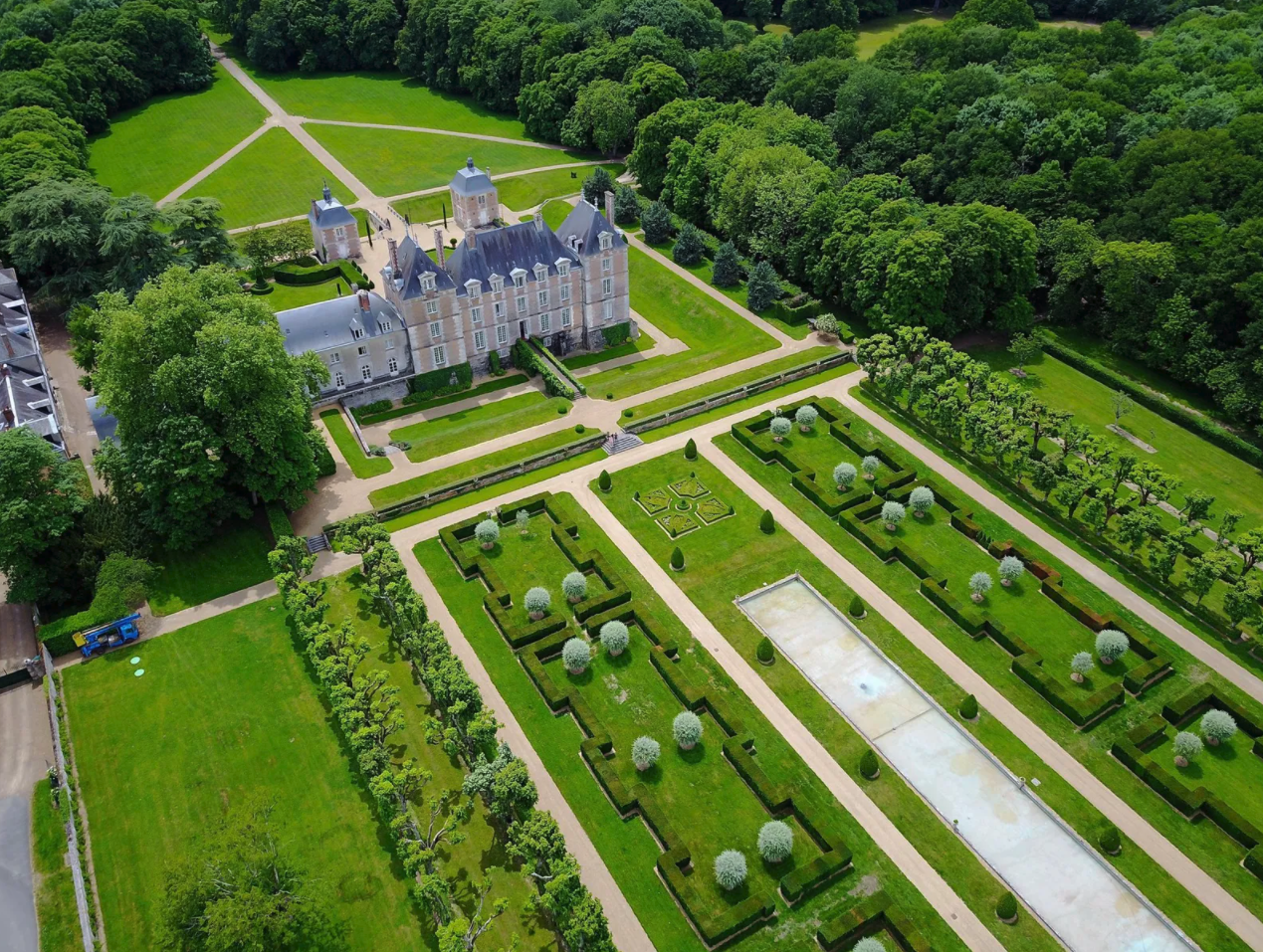This aerial view captures a grand, French-style palace surrounded by meticulously maintained gardens and lawns. The palace itself stands out with its dark gray roof and beige facade accented by white window trimmings. The layout includes rectilinear pathways and a rectangular fountain, creating a symmetrical and organized aesthetic. Large, lush green trees densely encircle the property, contrasting beautifully with the immaculately manicured hedges and bushes arranged in pairs throughout the gardens. Additionally, there's a distinct blue truck and another outbuilding partially visible to the left of the main structure. The overall palette of the scene features various shades of green, beige, gray, and touches of blue, adding to the visual richness and elegance of the landscape.